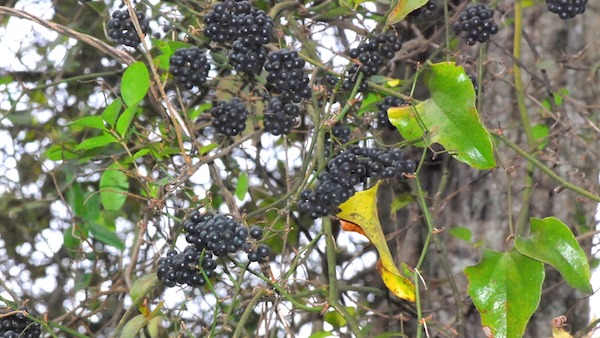This is a detailed close-up photograph of numerous small, round, black berries growing in dense clusters on a vine intertwined around a large tree. The berries, each resembling tiny globes akin to marionberries, form about a dozen distinct bunches, with clusters ranging from 15 to 20 berries each. They are the focal point of the image, appearing vibrant and inviting against the bright backdrop.

The vine features two different types of leaves: smaller, darker oval leaves and larger, waxy, triangular green leaves, with a hint of yellow found at the bottom of the image. The tree's rough gray bark occupies approximately the right third of the photograph, while the left two-thirds show a bright, possibly overexposed white sky, suggesting daylight shining through a dappled canopy.

Overall, the tree trunk is slightly blurred in the background, enhancing the sharp focus on the berries and leaves. The arrangement of the vine and the diverse leaves wrapping around the tree, alongside the scattered sunlit patches and the clear, photorealistic detail, convey a lively and textured natural scene.